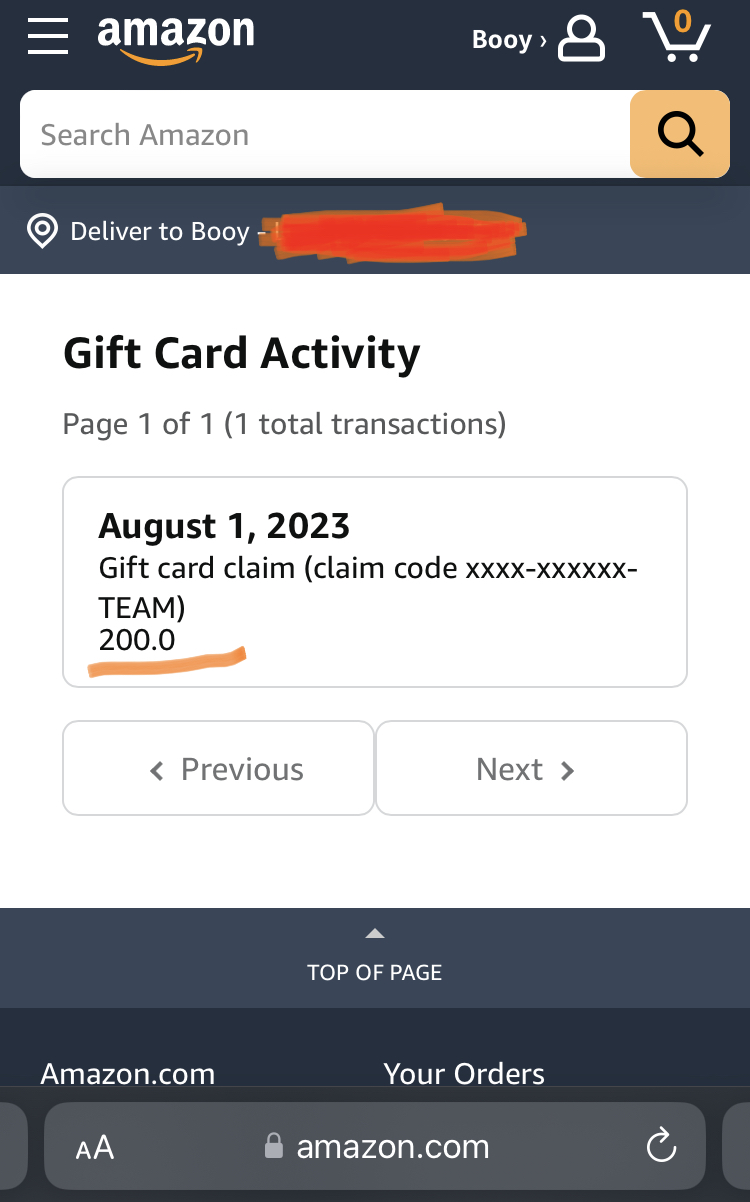The image is a screenshot from the Amazon website on a smartphone. At the top, there is a blue navigation bar featuring a white Amazon search box in the center. Above the search box, the Amazon logo is displayed in white letters with the iconic yellow smile arrow underneath it. To the right of the search box, the text "B-O-O-Y" followed by a right arrow is visible along with icons of a person and a shopping cart, the latter showing a count of zero items.

The search bar is empty except for the placeholder text "search Amazon." Below the search bar, the text "deliver to B-O-O-Y" is displayed, though part of this section is obscured by red ink. Further down, on a white background, the phrase "gift card activity" is prominently shown in black lettering. Beneath this, in smaller, lighter-colored text, it reads "page one of one" in parentheses and "one total transactions."

A detailed box follows, also on a white background with black text. At the top of this box, it says "August 1, 2023," followed by the text "gift card claim" and an obscured claim code. The amount "$200.00" is stated at the bottom of this section, underlined by what appears to be a line generated by a computer program.

Below this, two white boxes with gray lettering are displayed: one on the left labeled "previous" and one on the right labeled "next." Additionally, there is a dark-colored box that seems out of context, labeled "top of page" with a URL space containing "Amazon.com." This element appears to be misplaced as it does not align with the content displayed above.